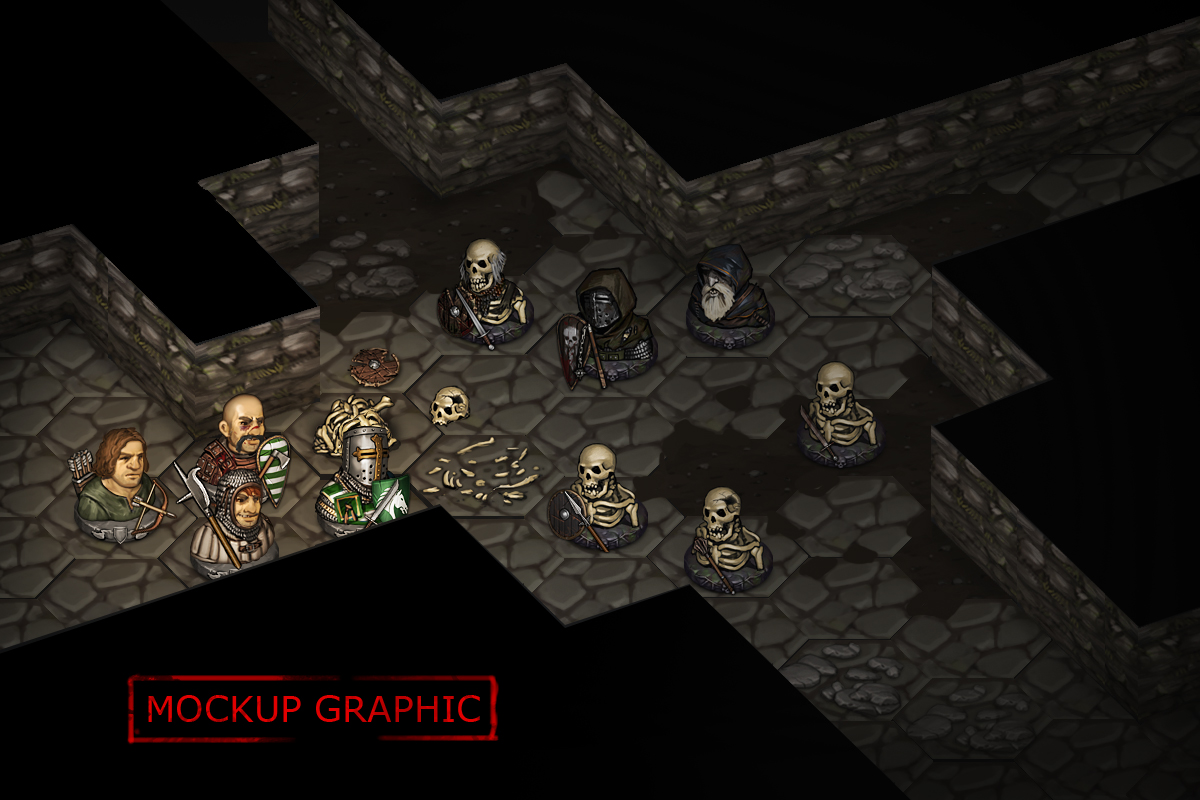The image appears to be concept artwork from a video game, depicting a dark, dungeon-like setting with a black background and a gray, stone-like floor. Central to the scene are various human warriors and skeleton figures, all seemingly emerging from the ground, as if they were game pieces attached to circular bases, resembling those in a physical board game. On the left side, four detailed human-like characters don armor and wield a variety of weapons: one with a bow and arrow, one with a staff, one holding a shield, and another clad in a helmet. These figures are arrayed against five skeletons or Grim Reaper-like figures equipped with swords and shields. A dismembered skeleton lies scattered on the floor, adding to the macabre ambiance. The bottom left corner features a red rectangle with the words "mock-up graphic" written in vivid red text, possibly indicating that this image is a preliminary design or a placeholder in the game's development process.